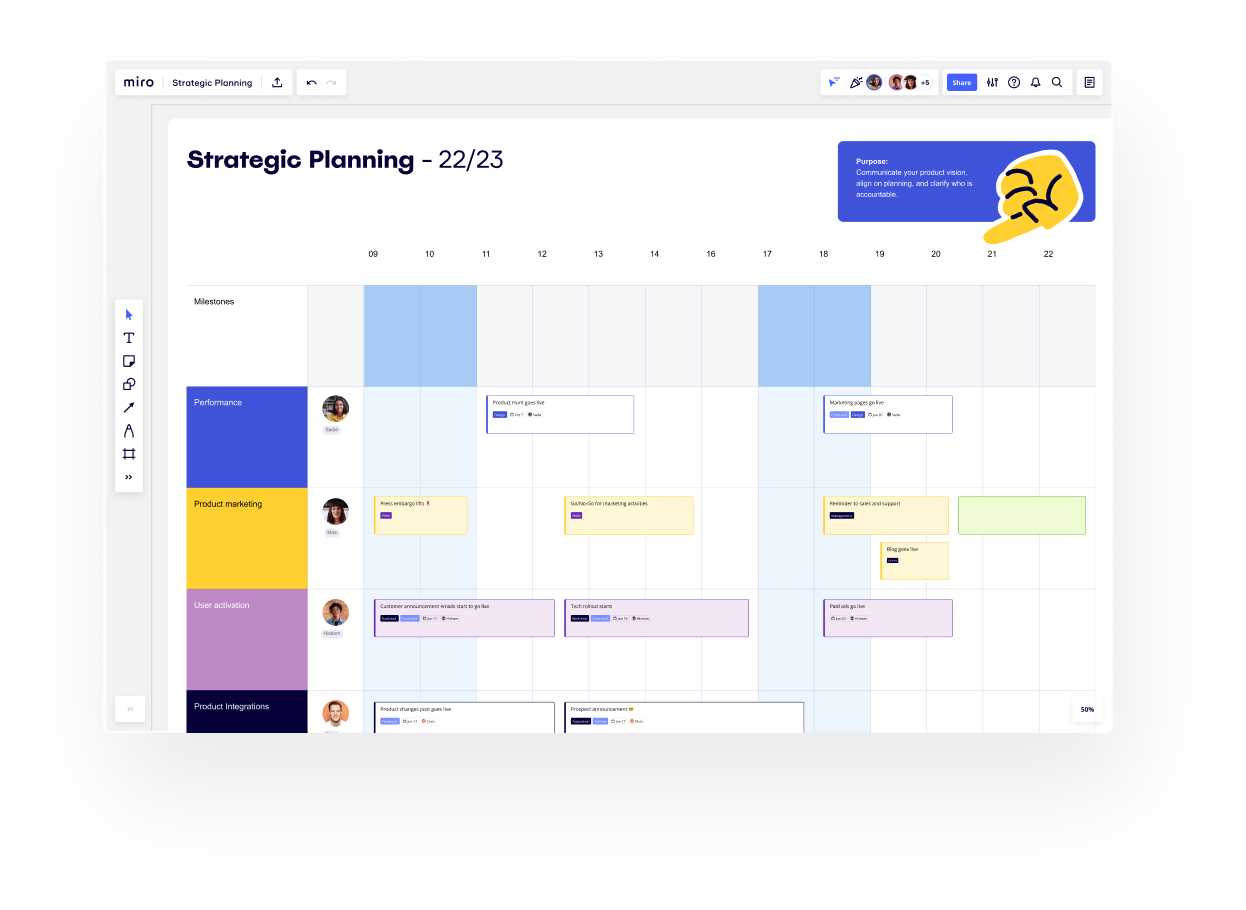This image is a detailed screenshot of a digital calendar or planning application, likely Miro, focused on strategic planning for the year 2022-2023. The interface features a gray navigation bar along the left side and across the top. At the top, the heading reads "Miro Strategic Planning." Beneath, the calendar grid is arranged by individual days, segmented further by hours, allowing for meticulous daily planning.

To the left of the calendar grid, there are several colored boxes used for organizing tasks or categories; these boxes are blue, goldenrod, lavender, black, and others are visible but partially obscured, suggesting the need for scroll navigation to view the content in its entirety. Unlike previous instances where content may have been cut off, this layout indicates the planner extends beyond the visible portion of the screen.

In the top right corner of the interface, there is a notable blue button featuring a yellow hand icon pointing downwards, perhaps highlighting a function or an initial instruction to start planning by selecting a date.